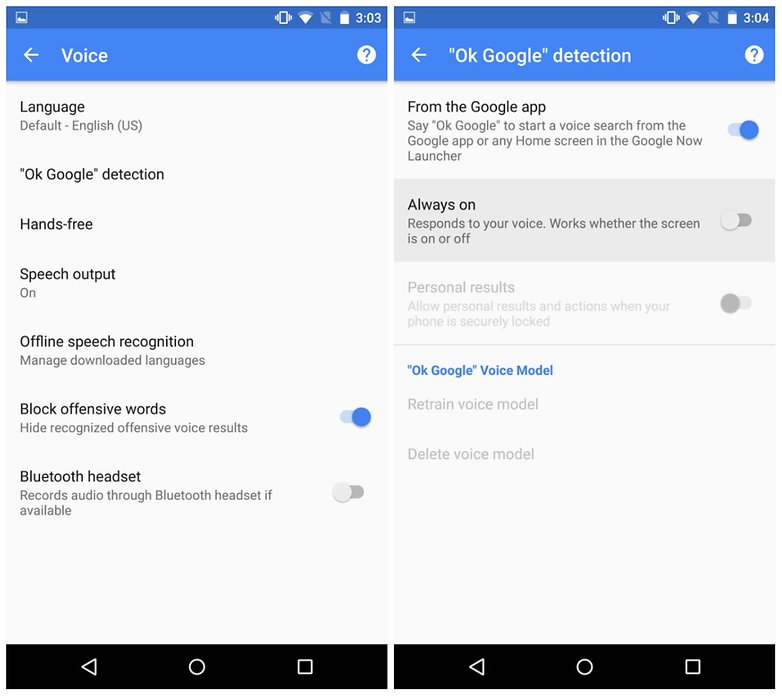The image consists of two side-by-side screenshots from a mobile device's settings pages focused on voice settings related to the Google app.

**Left Screenshot: Voice Settings Page**
- **Header:** Blue with the title "Voice"
- **Settings Below:**
  - **Language:** Set options
  - **"OK Google" Detection:** Configuration options
  - **Hands-Free:** Manage hands-free options
  - **Speech Output:** Currently switched ON
  - **Offline Speech Recognition:** Available settings
  - **Block Offensive Words:** Currently switched ON
  - **Bluetooth Headset:** Currently switched OFF

**Right Screenshot: "OK Google" Detection Page**
- **Header:** Blue with the title "'OK Google' Detection"
- **Settings Below:**
  - **From the Google App:** Switched ON
  - **Always On:** Displayed within a gray rectangle, currently OFF
  - **Personal Results:** Currently OFF
  - **"OK Google" Voice Model:** Options to retrain or delete the voice model

The background of both pages is white with a straightforward layout of settings in black text, enhancing readability and ease of navigation.